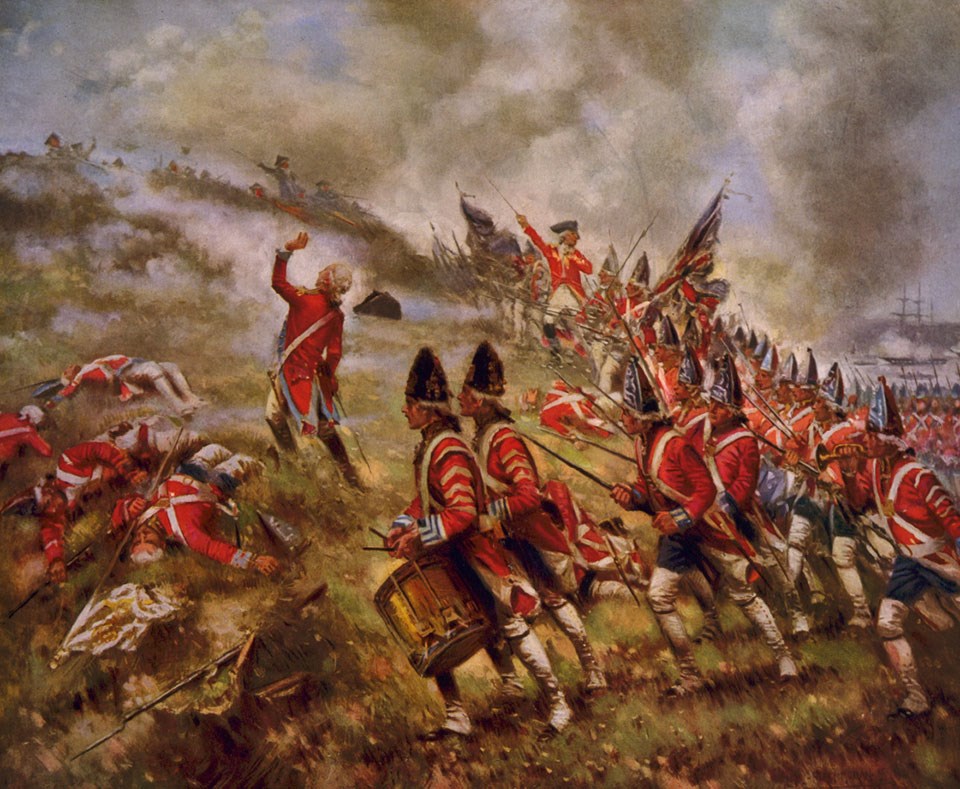This detailed historical painting depicts a battle scene set on a grassy hill. The primary focus is on the British soldiers, identified by their distinctive red coats, dark-colored pants, and white lower leggings. They are advancing from the right side of the image toward the top left, where the hill's summit is visible. These soldiers are equipped with various weapons, including swords and rifles with bayonets. Many wear tall pointy hats, adding to their distinctive appearance.

In the lower center of the image, a soldier wearing a pointed hat and playing a drum stands out among his comrades. Close to him, in the lower left, there are four dead soldiers lying on the ground, one of whom holds a white flag, symbolizing surrender or a call for a truce.

Near the center left, halfway up the hill, the leader of the British troops is captured in the midst of motion, his arm extended upward as if urging his men forward toward the hilltop. The background of the painting is rich with additional details, including ships in a distant harbor, signifying a wider context of warfare and conflict. Smoke clouds the air, adding to the chaotic atmosphere of the scene. This evocative painting encapsulates the intensity and complexity of historic battles, with hundreds, if not thousands, of soldiers depicted in an epic clash that resonates with the brutal realities of war.